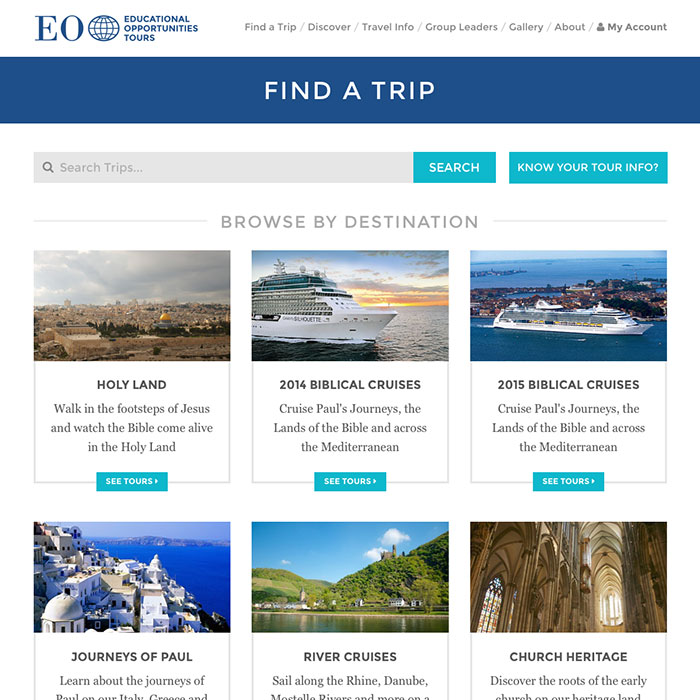On a white background, the website header features menus with text in dark gray, including "Educational Opportunities," "Tours," "Find a Trip," "Discover," "Travel Info," "Group Leaders," "Gallery," "About," and "My Account." Prominently displayed is a blue rectangle with "Find a Trip" in white text. Below, there's a search bar labeled "Search Trips" with a magnifying glass icon and a blue "Search" button featuring white text.

The page encourages users to "Know Your Tour Info" on a blue rectangle. In a section labeled "Browse by Destination," six key destinations are highlighted. First on the list is "Holy Land." Adjacent is another blue rectangle labeled "Sea Tours," showcasing options like "2014 Biblical Cruises" and "2015 Biblical Cruises," each accompanied by informative details. Additional sections include "Sea Tours," "Journeys of Paul," and "River Cruises," each offering specific information. Under "Church Heritage," the site invites users to "Discover the roots of the early church on our heritage land."